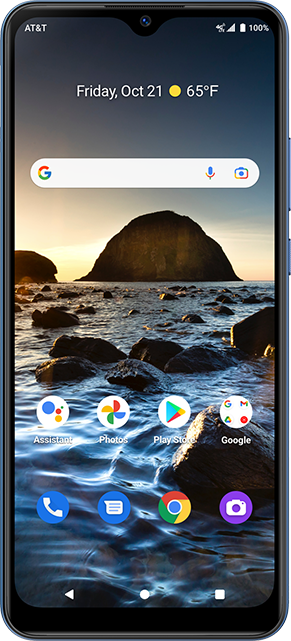The image displays a smartphone with visible bezels and side buttons, showcasing its detailed home screen. The home screen features a dark, evening-themed ocean scene with a rocky shoreline and large, mountain-like rocks emerging from the water in the background, suggestive of a bay area. At the top of the screen, the date "Friday, October 21" is displayed alongside a small yellow sun icon and a temperature reading of "65°F." Centered towards the top is a Google search box, identified by a Google logo on the left and icons for voice and image search on the right. 

The lower part of the screen is populated with several shortcut icons: Google Assistant, Google Photos, and Google Play Store. An expandable quick launch drawer contains shortcuts for Gmail, Google Drive, and Google Music. Positioned at the very bottom of the screen are additional app icons for Phone, Messages, Google Chrome, and the Camera app.